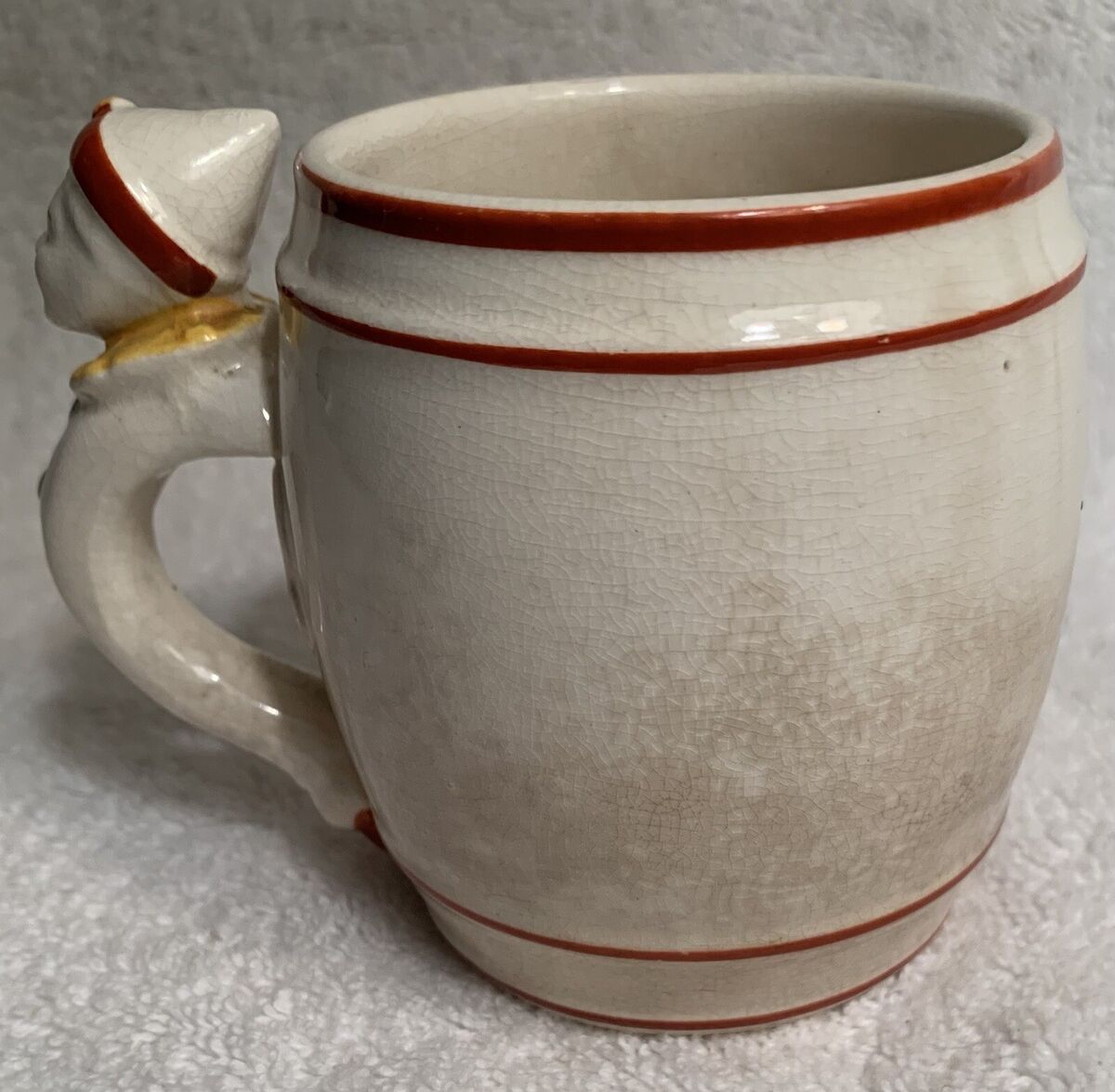The image is a tightly framed close-up of a cherished, ceramic coffee cup, filling the entire frame. The cup, which is a beige or white color, bears signs of age and use, with a cracked glaze pattern covering its surface. It features two decorative maroon or burgundy bands around its top rim and a second set of bands near the base. The most striking element is the handle, an ornate piece shaped like a small boy or elf wearing a hat. This figure is also the same beige color, with the hat adorned by a matching maroon or burgundy rim. There is noticeable discolored beige glue where the head had been reattached to the handle, suggesting the cup has been repaired and is well-loved. The background reveals the cup is placed on a gray carpet or some sort of flooring, which almost matches its color, creating a harmonious visual blend.